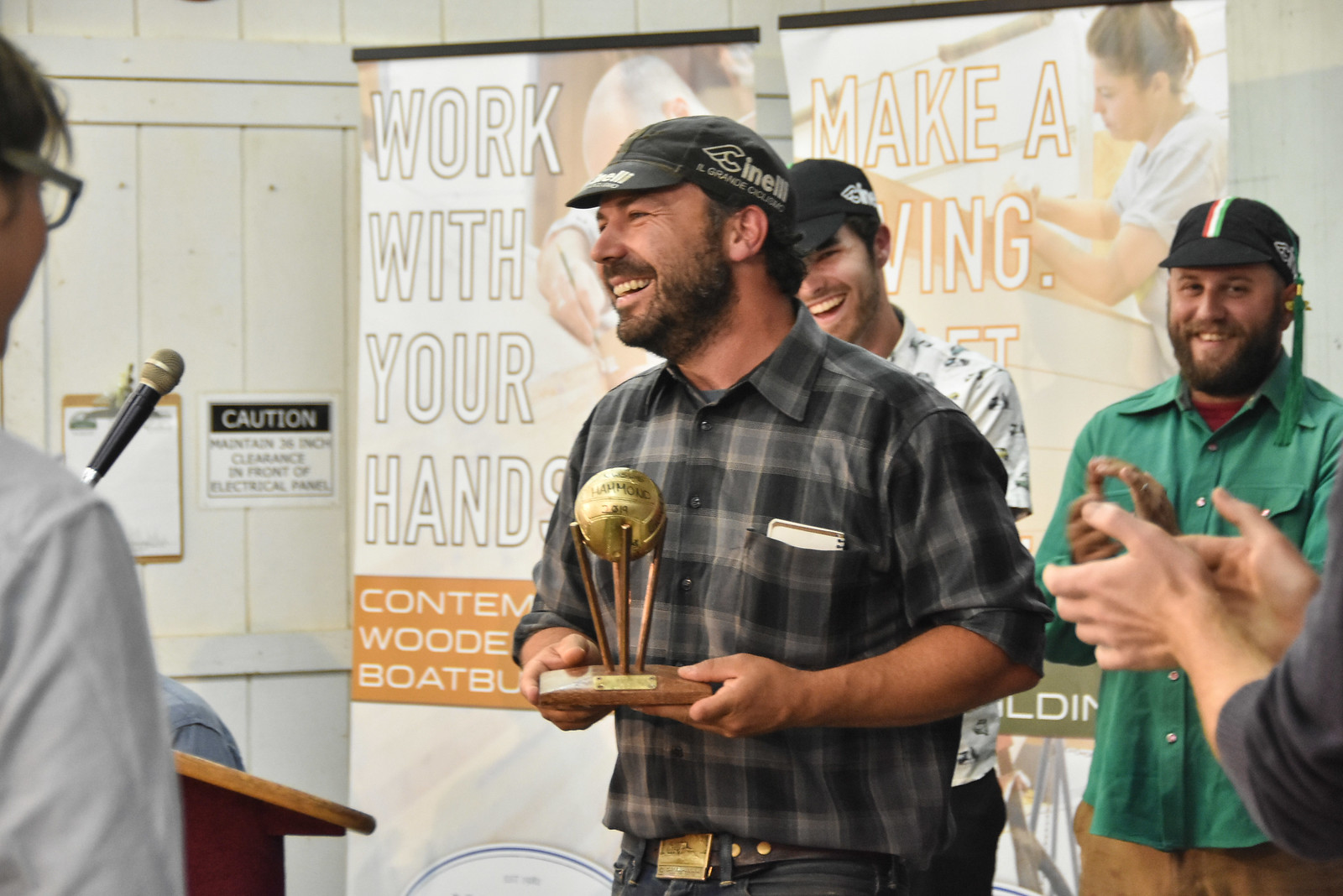In the photograph, a bearded man, dressed in a black and gray checkered shirt, black hat, and blue jeans, stands at the center holding a distinctive golden trophy. The trophy features a ball, resembling a volleyball or soccer ball, supported by four sticks on a wooden base. He is smiling and looking slightly to the left while cradling the award with both hands. The man's shirt pocket is adorned with a notebook. Surrounding him, people are applauding and smiling, suggesting a celebratory atmosphere. In the background, two banners are visible, one clearly stating "work with your hands" and the other partially obscured with "make a living." A podium with a microphone stands to the bottom left of the image, and an individual is also seen standing to the left. The setting appears to be indoors with white walls.